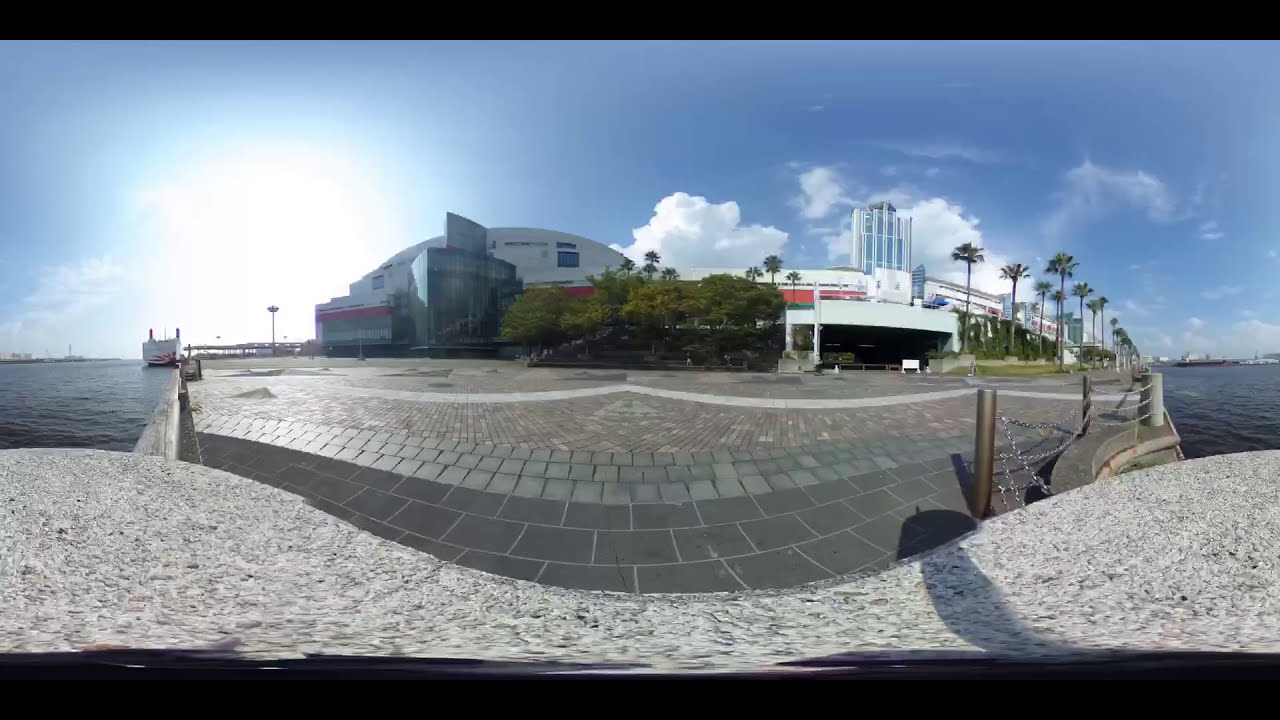The image captures a picturesque waterfront scene featuring a large, elegant building extending into a body of water, likely a harbor or port. The structure, which seems to serve a commercial or observational purpose, is painted in white, blue, and red, with prominent design elements suggesting modern architecture. Surrounding the building, lush greenery includes palm trees and other verdant foliage, adding a tropical ambiance to the scene.

The foreground consists of a cobblestone and concrete pavement, accompanied by chain-link fencing, creating a robust yet accessible pathway. The pavement appears to lead directly to the building, resembling a wide pier jutting out into the water, suggesting an integration with its maritime setting. One can spot a boat on the left side of the image and possibly other watercraft to the right, enhancing the nautical atmosphere.

The background reveals a tall tower which could be associated with logistical functions like a parking structure or a delivery drop-off spot, signaling the building's functional versatility. The absence of people and the presence of shadows cast by intermittent clouds provide a serene, almost untouched quality to the photograph. It's suggested that the location could be something notable like the Rose Bowl in Pasadena, California, though it looks distinctly more like a docking site or a business headquarters near a coastal area. The sky, punctuated with a few clouds, completes the tranquil and expansive view.